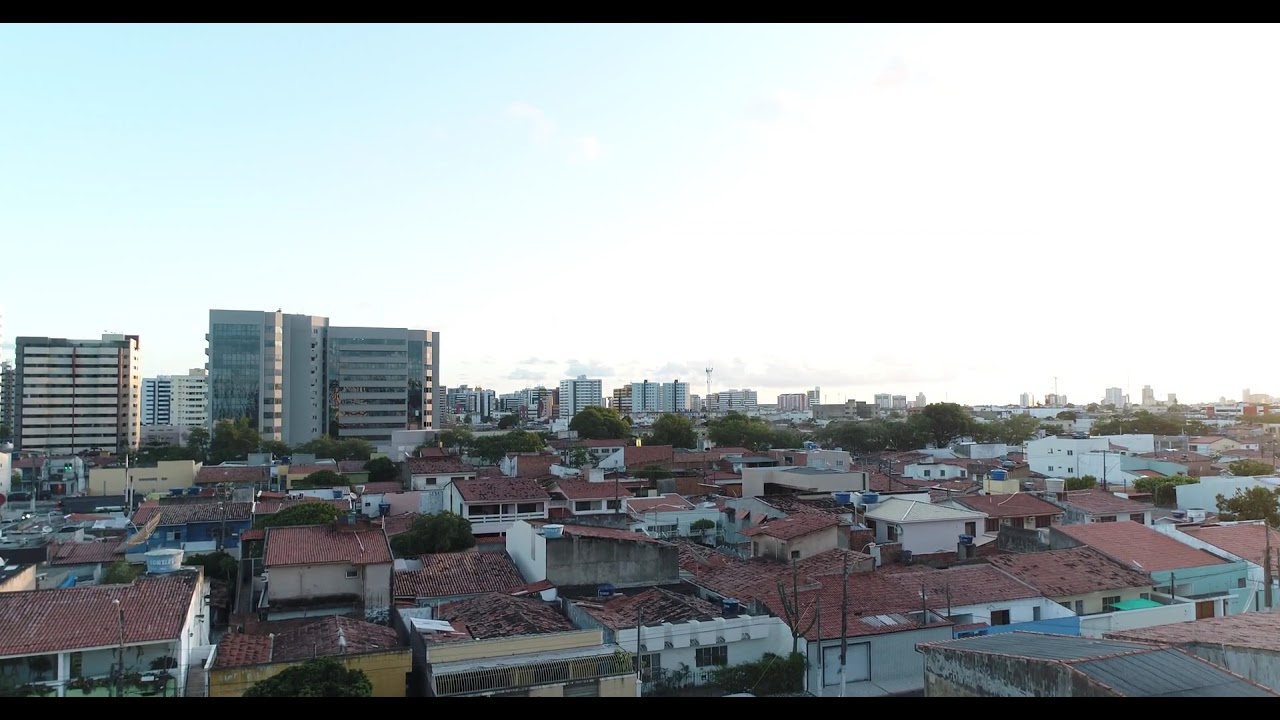The image is a panoramic view of a city captured from an elevated vantage point. The lower half of the photograph is densely populated with an abundance of one- and two-story buildings, predominantly featuring red roofs. These smaller structures appear to be mostly residential, compactly arranged without visible lawns or open spaces. The buildings' colors range from dark blue to beige and yellow, creating a vibrant mosaic. Towards the horizon, about mid-way up the photograph, stand several tall, rectangular skyscrapers on the left, gradually receding into the background. The upper half of the image is dominated by a bright sky, transitioning from a sun-soaked white near the horizon to a deeper blue as it ascends. The sky is interrupted by a long, white cloud stretching horizontally. Overall, the image beautifully contrasts the compact residential area with the imposing skyline and expansive sky above.